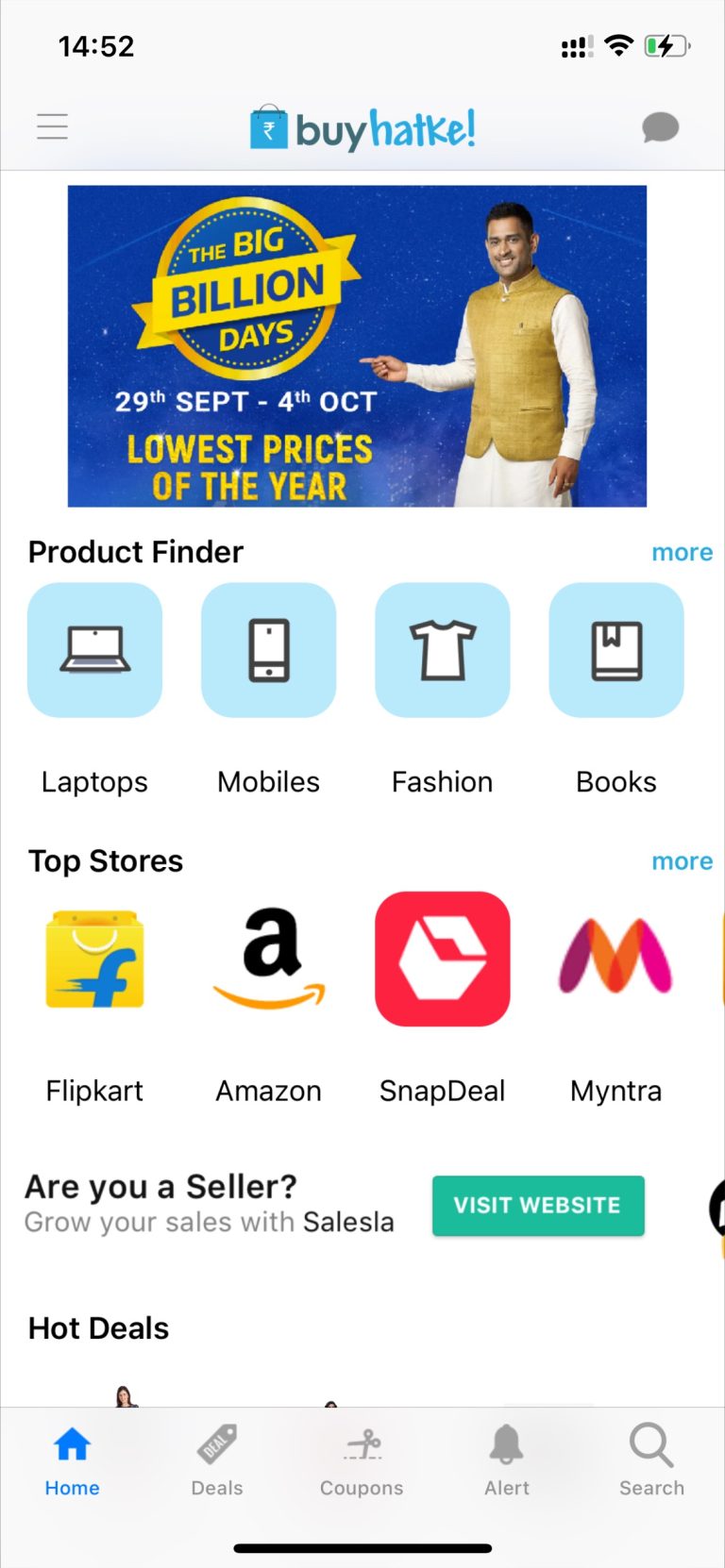This is a detailed caption for the given image:

---

This image is a screenshot captured from either a mobile app or a website, displayed on a smartphone. At the very top of the screen, the time is shown as 14:52, accompanied by typical phone icons indicating notifications and signal strength. The header banner of the application or website is branded by "Hotkey" (H-A-T-K-E).

Beneath the header, there is a prominent promotional banner featuring an image of a man dressed in a long white shirt and a gold vest, pointing towards the text of the banner. The banner advertises "The Big Billion Days," scheduled from 29th September to 4th October, highlighting it as the period with the lowest prices of the year.

Below the promotional banner, the interface features a section titled "Product Finder," which includes four blue boxes with white icons and text that categorize different product types: 
1. Laptops
2. Mobiles
3. Fashion
4. Books

Following this section, "Top Stores" are listed with their corresponding logos: Flipkart, Amazon, Snapdeal, and Myntra.

Further down, there is a segment addressing sellers with the text: "Are you a seller? Grow your sales with Sales Slot," accompanied by a green button labeled "Visit Website."

The bottom section of the screen showcases "Hot Deals," and a navigation bar with five icons and labels: 
1. Home (with a blue home icon)
2. Deals
3. Coupons
4. Alert
5. Search

This organized layout summarizes the key features and promotional content of the app or website.